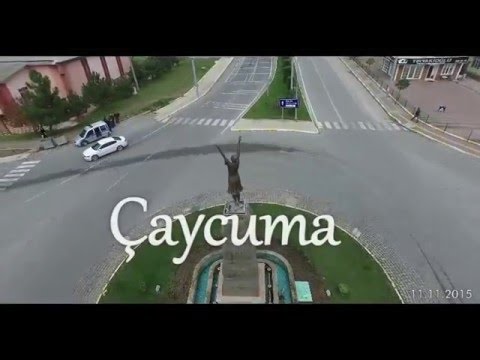The image captures an aerial view of a bustling roundabout, prominently featuring a large statue of a young woman with her arms raised toward the sky, situated on a tall stone pillar in the center. Surrounding the statue is a well-maintained grassy area encircled by a circular street, indicating the roundabout. The scene is adorned with vivid colors including gray, white, green, blue, black, and pink, with noticeable text at the bottom reading "Kei Kuma."

Visible on the left side of the image are a few vehicles: a white car making a right turn towards the left side of the image, and a gray van parked by the roadside. There are buildings on both the top left and top right, with a distinct red-pink building on the left. The right part of the image, near the bottom corner, features a person walking on the sidewalk and a crosswalk. The roundabout is framed by two lanes of traffic separated by another grassy divider, with trees in the background contributing to the outdoor setting. Additionally, a date noted in the lower right corner reads November 11th, 2015, providing temporal context.